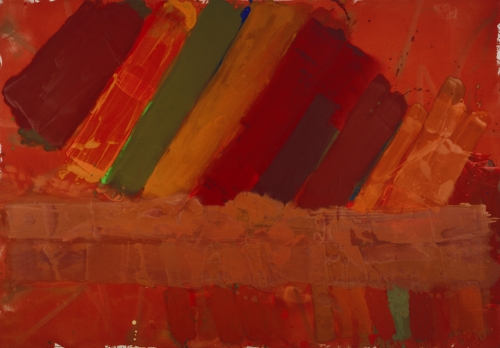This abstract modern painting, rendered primarily in shades of red and burgundy, features a striking interplay of vertical, horizontal, and diagonal elements. The bottom half of the small, horizontal rectangular image showcases a rough, almost brick-like surface with occasional streaks of green. Above this textured lower section, a series of slanted, pillar-like forms in various shades of red and burgundy extend diagonally from the bottom left to the upper right, giving the impression of leaning books. Between these prominent, slanted forms, there are both darkened areas suggesting shadowy pillars and vibrant patches of green, similar to the streak below, adding contrast. The overall composition includes a blend of orangish and maroon hues, creating a layered depth within the chaotic yet harmonious arrangement of shapes and colors.